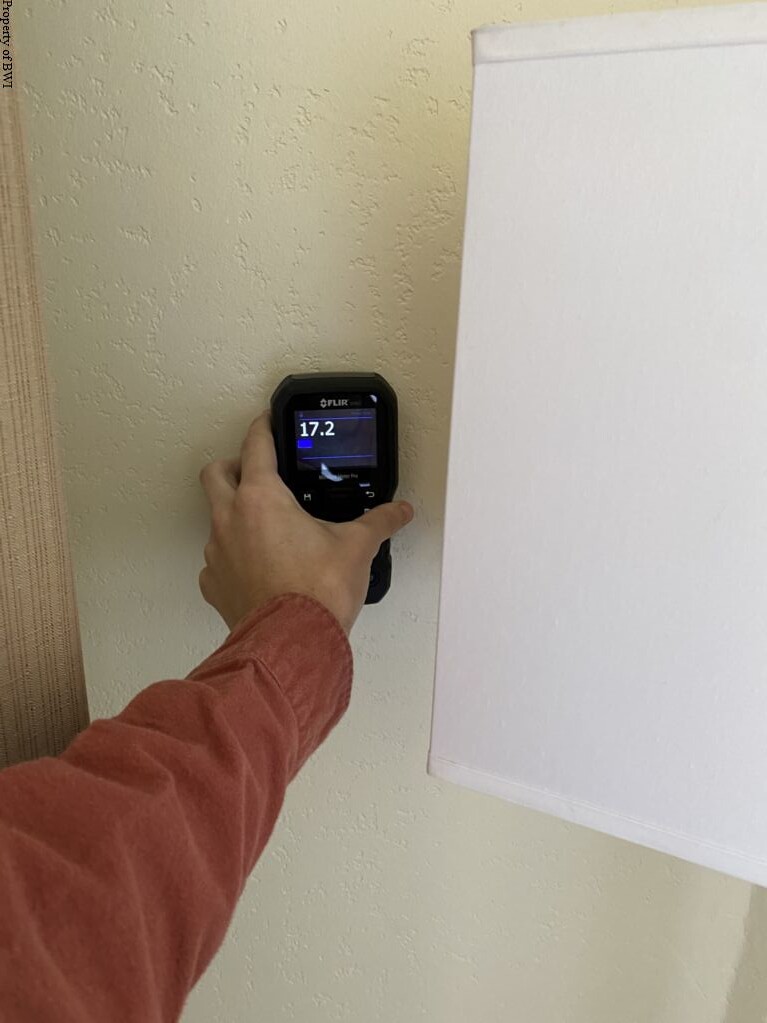In this high-quality photo, a person's hand is seen pressing a black FLIR device against a tannish-colored wall. The device displays the reading "17.2" on its screen, suggesting it is measuring some attribute of the wall, potentially temperature or thickness. The hand enters the frame from the bottom left corner, firmly grasping the device. To the left of the image, a bit of a curtain is visible, adding a touch of fabric texture to the scene. On the right side, a large white, rectangular shape, likely a lampshade, is partially in view. The device itself features several buttons; a return button is clearly visible, alongside another button marked with the letter "H". The remaining buttons are obscured by the user's hand. This detailed setup suggests a careful and precise measurement is taking place.